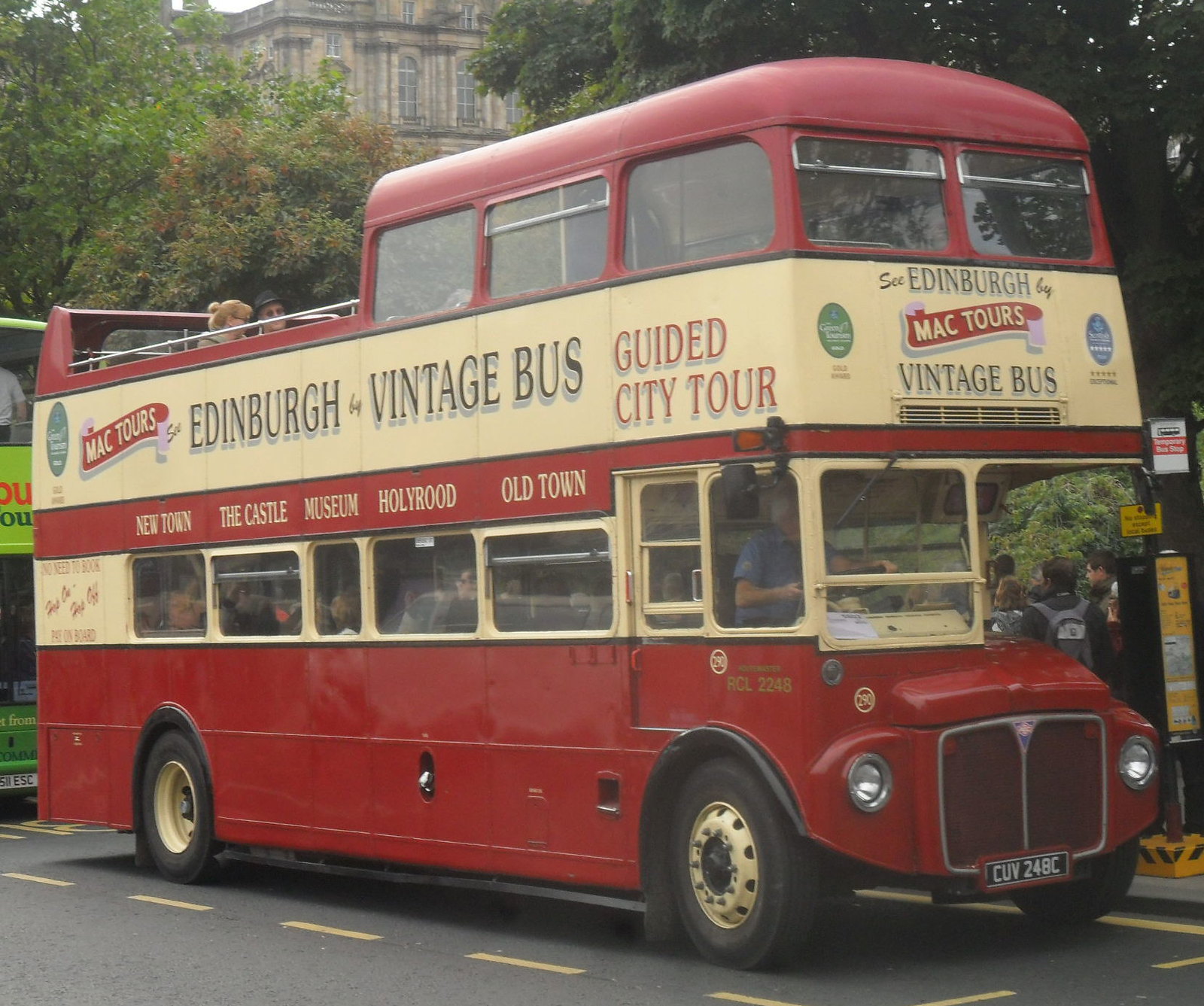This image features a vintage red double-decker bus, distinguished by its classic design reminiscent of the 1960s. The bus has been converted into a tour bus operated by "Mac Tours," offering guided city tours of Edinburgh. The bus sports cream-colored bands around the windows and a beige base on the top part, contrasted with red areas bearing white and red text. Prominently displayed on the bus are the phrases: "Mac Tours Edinburgh Vintage Bus," "Guided City Tour," and a list of the destinations covered—Newtown, The Castle, Museum, Holyrood, and Old Town. The top deck has an open-air section towards the back, where a man in a black hat and sunglasses sits beside a blonde woman with her hair in a bun. The front half of the upper deck is enclosed with a red roof, while the driver is visible in the front driving compartment. The street scene also shows numerous people waiting at the bus stop, highlighting the popularity of this picturesque tour through Edinburgh’s historic sites.